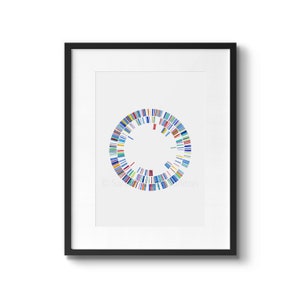The image is a color photograph of a framed piece of artwork hanging on a white background. The frame itself is thin and black, casting a shadow on the right side and bottom portion. Inside the frame, a white border surrounds the artwork, which sits on an off-white or very light gray background.

The centerpiece of the artwork features a series of three concentric circles. These circles are composed of numerous narrow rectangular slits of various colors arranged side by side. The outermost circle is densely packed with colors, including blues, reds, yellows, greens, purples, oranges, pinks, browns, blacks, and teals. The middle circle has fewer color slots and appears more sparse. The innermost circle is the most incomplete, with large gaps between the few remaining colored slits, predominately showcasing a white background. Overall, the concentric circles create a vibrant and varied display, representing nearly all colors of the rainbow but growing sparser towards the center. There is no indication of the artist or title of the piece within the image.